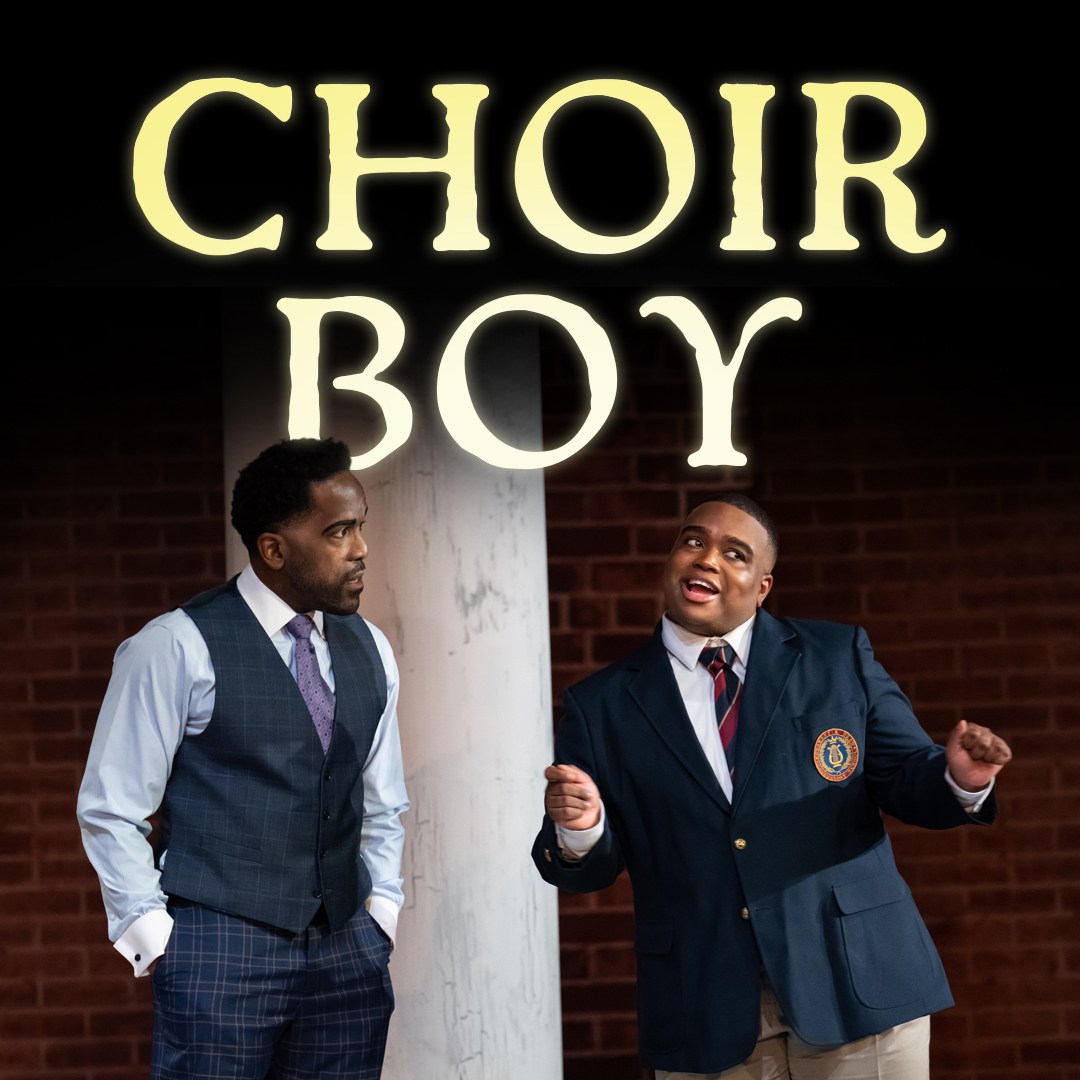The image appears to be a poster for a movie or show titled "Choir Boy," as indicated by the yellow to white gradient text at the top of the poster, which fades from black to reveal the image. The background features a red brick wall and a white cement column. The poster prominently displays two African-American men. The younger man, likely a student, is dressed in a dark blue school uniform jacket with a white button-up shirt and a blue-red striped tie, along with tan pants. He is smiling and animated, tilting his head while making a side-eye gesture with his hands in a fist. To his left is an older man, possibly in his late 30s or 40s, who may portray a principal or an administrative figure. He is dressed in professional attire, featuring a plaid vest, light blue and white button-up shirt, purple patterned tie, and plaid pants. The older man looks at the younger one, possibly with a judgmental expression.